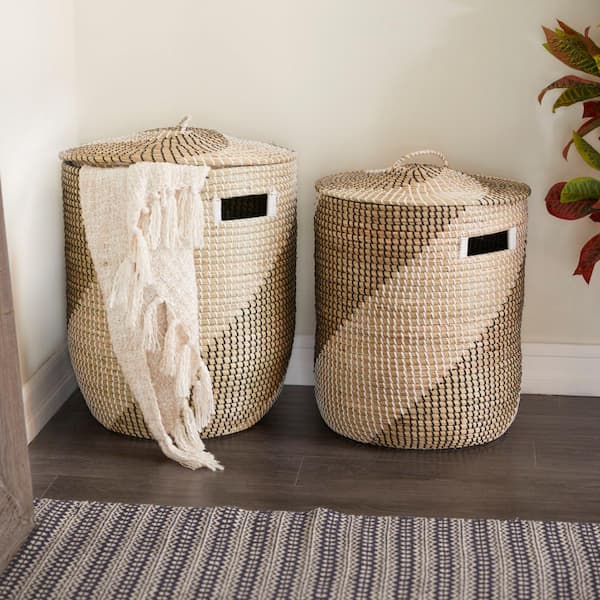The image depicts the cozy corner of a room, showcasing two woven, beige-colored jute laundry hampers, placed side by side. The larger hamper is on the left and has a white piece of fabric, which appears to be either a blanket or shawl, protruding from under its canvas-like lid. Both hampers share the same cylindrical design with diagonal light white straps running across the middle, and feature black slits below the lids for easy handling. The room's walls are painted a light cream color, accented by white floor molding. There's a hint of greenery with green and red leaves from a plant on the right side. The floor below the hampers is covered by a dark brownish-gray hardwood, partially overlaid with a thin rug displaying dark gray, light gray, and navy stripes. In the background, a door with a grayish-brown hue is slightly ajar.